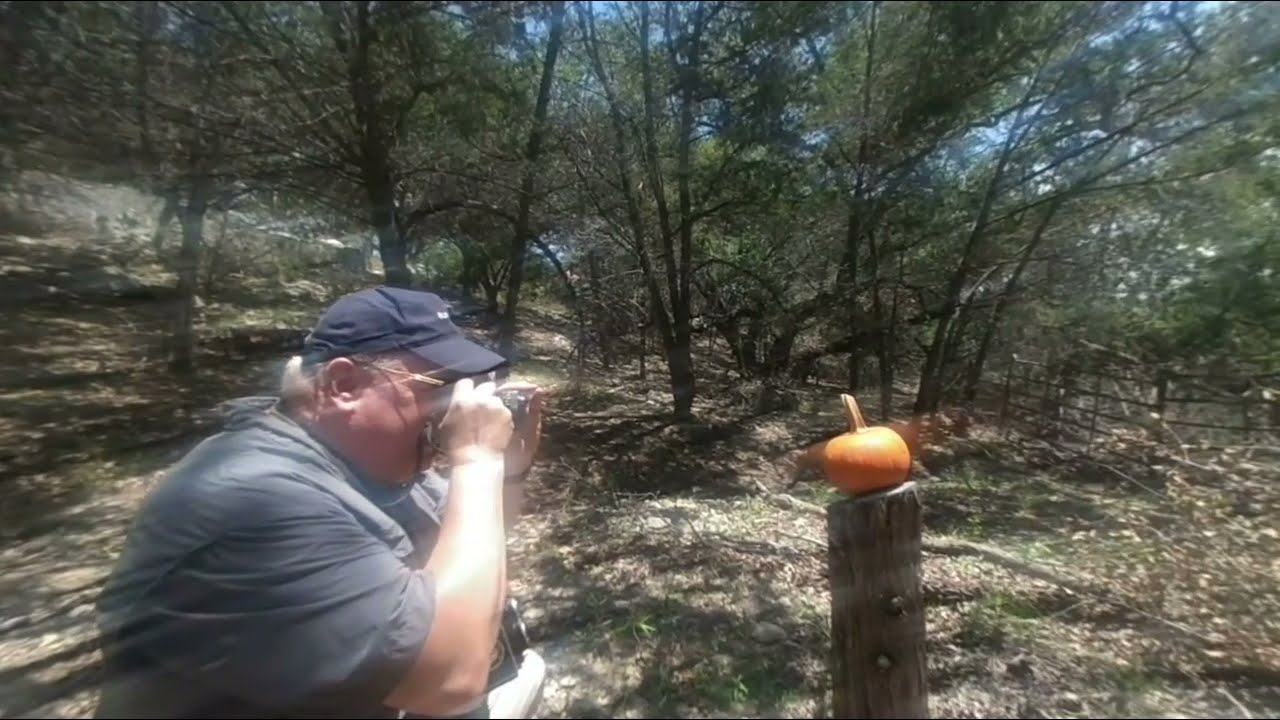In a sunlit, wooded area, a man with peach-colored skin is captured in the foreground, wearing a blue shirt, blue cap, and glasses. He is holding a camera up to his face, seemingly focused on taking a picture. Positioned to the lower left of the image, he directs his camera towards a small, vibrant orange pumpkin that rests upon a wooden post at the center right. The ground is a mixture of light brown and green, dotted with grass, dead leaves, and twigs, indicating the forest floor. Behind him, a patch of green trees rises, mingling with the blue sky peeking through the canopy. To the right, a steel fence subtly marks the boundary of this serene, rustic scene.